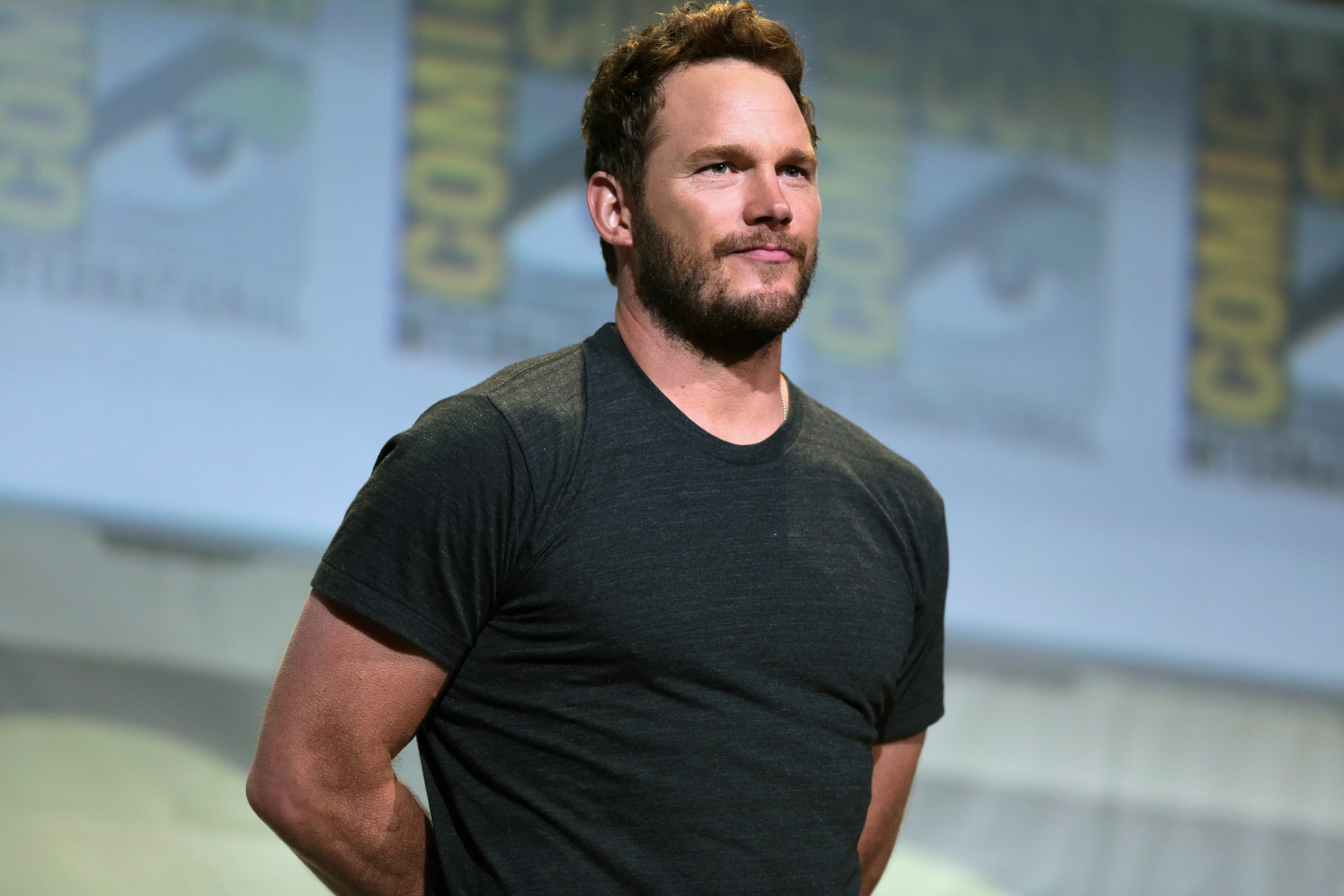This photograph captures a close-up of Chris Pratt standing indoors at Comic-Con. He is depicted from the waist up in a standing position with both arms held behind his back, his elbows visible. Chris is wearing a black, short-sleeve t-shirt and has neatly styled short brown hair that is slightly puffed up and swooped at the front. He sports a full beard that includes a mustache, which connects to his sideburns, and his skin is a fair complexion. Chris's facial expression shows a small smirk with his mouth closed as he looks straight ahead, likely at the audience in front of him. The background is blurred, featuring a repetitive Comic-Con logo along with some posters that have text in yellow. The lower half of the background includes a beige wall, adding to the convention setting atmosphere.